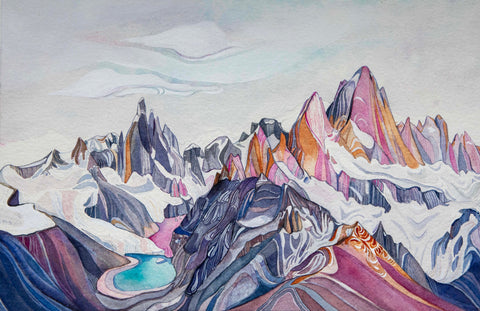This abstract painting, possibly created with colored pencils or watercolors, vividly portrays a mountainous landscape that is both colorful and striking. The snow-covered peaks are intricately detailed with sharp, jagged points that cascade downwards, creating an impression of multiple vertical layers of mountains in direct contact. These peaks are adorned with a palette of purples, dark blues, teal, violet, and dark greens, with hints of white or light blue used for shading. The left side of the image features a notable divot, which leads to a small, circular body of blue water surrounded by a sandy area. The sky above is a light, hazy blue or gray, dotted with a few clouds, offering a stark contrast to the vibrant mountains below. Despite the intense coloration of the mountains, the sky maintained a subdued tone. The painting is wider than it is tall, and there are no signs of human presence, signatures, or watermarks, leaving the viewer to focus solely on the captivating, abstract mountainous scenery.